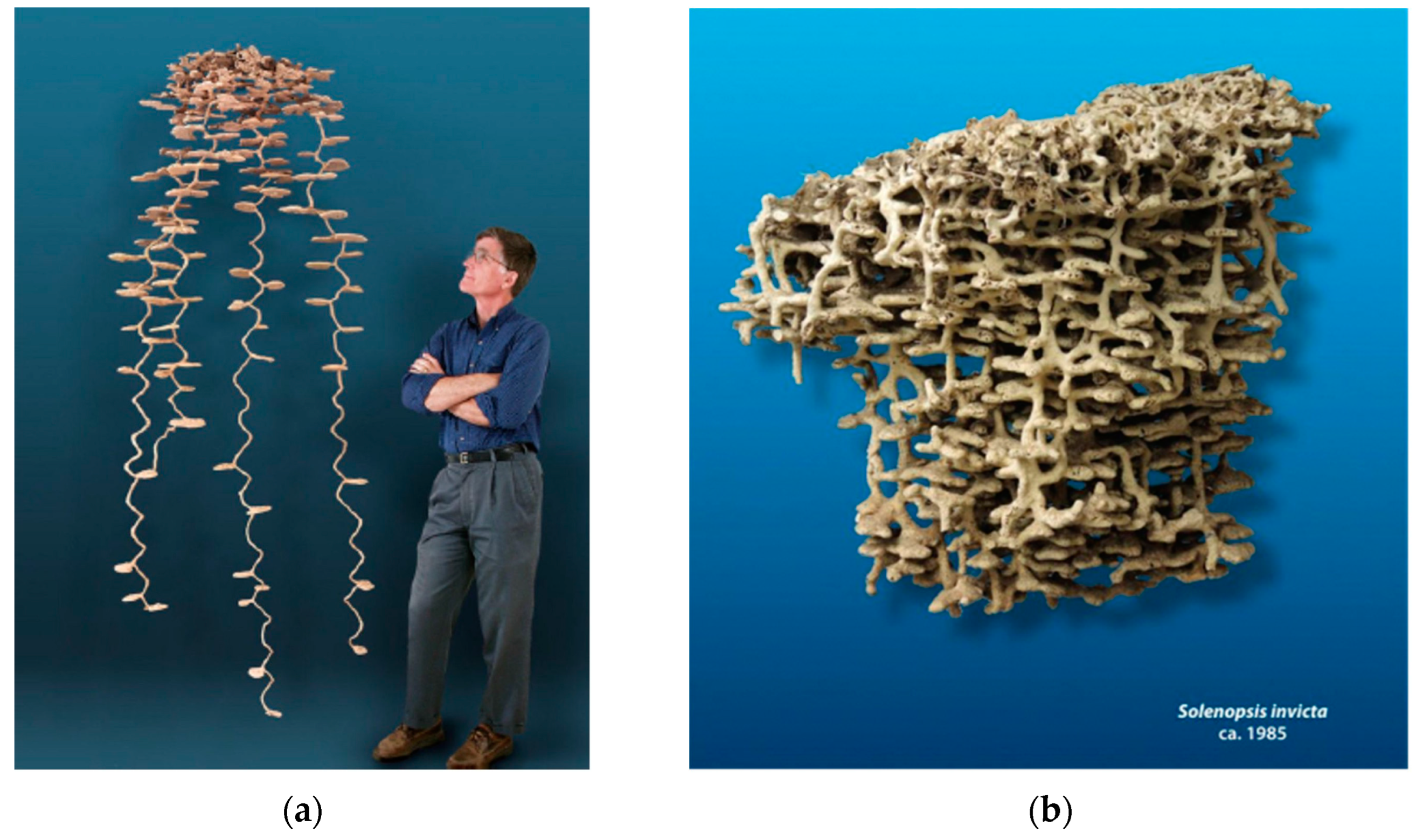The two side-by-side photographs displayed on a white background both feature a turquoise blue backdrop. In the left image, labeled with "(A)", a man stands on the right side, observing an intriguing object overhead. The man is dressed in a long-sleeved blue button-up shirt, gray pants, a black belt, brown shoes, and glasses. With arms crossed, he gazes up at what appears to be an intricate cluster of tan, light brown, and dark brown strands. The cluster, positioned well above the man, has several strands hanging down—one long strand to the left, a shorter one next to it, the longest strand in the center-right, and another long one closest to the man. 

On the right side, the photograph labeled with "(B)" provides a close-up of the mysterious structure. The mass looks similar to pathways created by ants and bears a resemblance to a catacomb or honeycomb pattern, with strands of grey, tan, and brown intertwining and intersecting on a turquoise blue background. The structure is denser at the top and gradually thins out as it extends downward. Additionally, the label "SOLENOPSIS INVICTA" is visible at the bottom right, along with "CA. 1985," indicating that the image likely represents the intricate tunnel systems formed by the Solenopsis invicta ant species.